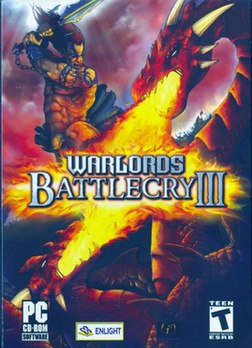The image depicts a stock photo of the PC CD-ROM game case for "Warlords Battlecry 3." Dominating the cover is a dynamic scene featuring a fierce battle between a barbarian warrior and two dragons. The warrior, heavily muscled and clad in a loincloth, exudes a barbaric strength as he leaps into the air, wielding a sword that is also chained to his arm, poised to strike. He is adorned with tribal tattoos or chains that accentuate his wild appearance. His hair is a fiery red, matching the intensity of the scene.

To his right, a formidable dragon unleashes a torrent of fire, its menacing presence captured in the fiery red hues of its scales. On the bottom left of the cover, another dragon mirroring the first, also breathes fire, with both streams of flame converging in the center of the image, producing a dramatic effect. This fiery meeting point is strategically placed behind the bold, stylized text "Warlords Battlecry 3."

The background of the cover is suffused with deep red tones, evoking the tumultuous atmosphere of a stormy battlefield. The fiery red and stormy clouds amplify the intensity of the scene, drawing the viewer into the chaos of the battle.

At the bottom left corner, the words "PC CD-ROM" appear, below which there is some unreadable text. Centrally at the bottom, the logo of the game publisher, "Enlight," is prominently displayed. Meanwhile, the bottom right corner features the "T for Teen" rating, indicating the game's appropriate age group.

This visually arresting cover art effectively captures the epic and dramatic essence of "Warlords Battlecry 3," promising an adventurous gaming experience filled with fantasy and combat.